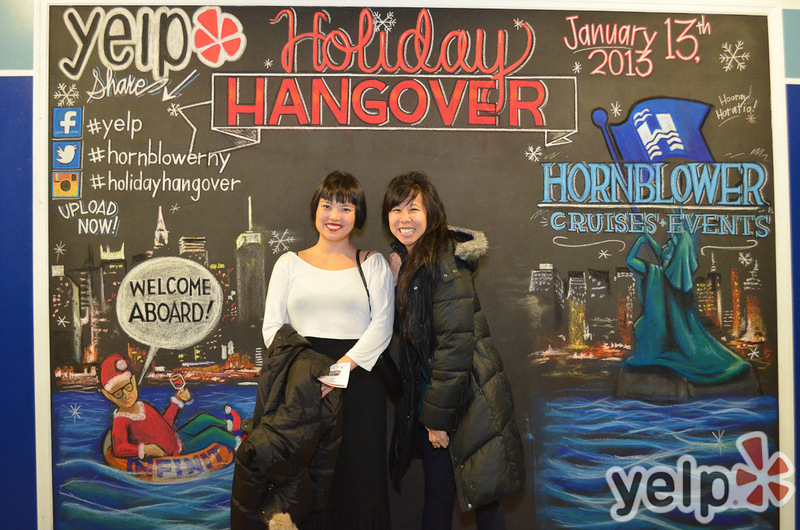In the image, two Asian women stand smiling in front of a detailed chalkboard sign. The sign, which has a white frame, features a city skyline with blue water at the bottom, and a black sky above. At the bottom of the scene, an elf dressed in green tights, a red shirt, and a Santa hat sits in an orange inner tube, with a speech bubble that reads, "Welcome aboard." The top of the sign includes red text that reads, "Holiday Hangover, January 13, 2013," with additional text promoting Yelp, Hornblower Cruises Events, and social media platforms such as Facebook, Twitter, and Instagram with hashtags #Yelp, #HornblowerNewYork, and #HolidayHangover. On the right side, there's an illustration of the Statue of Liberty holding a blue flag with a white "H" for Hornblower. Snowflakes are depicted falling from the sky. The woman on the right wears a long black puffer jacket and has long brown hair, while the woman on the left wears a white blouse and a black dress, with short black hair, holding a black puffer jacket.